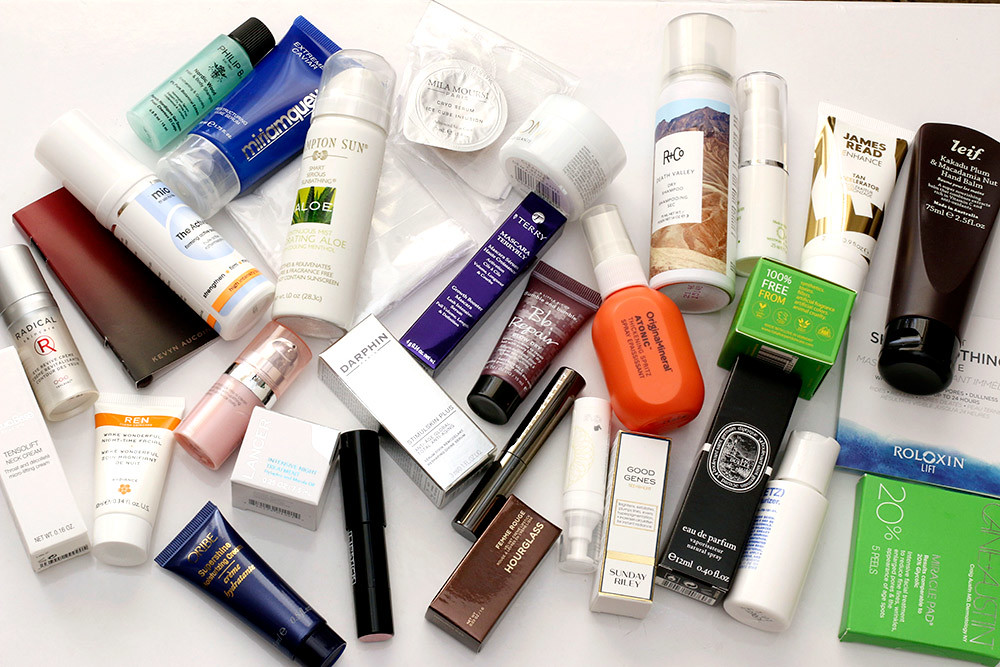In this image, an assortment of beauty products is meticulously arranged against a stark, white background. On the far left, a colorful box labeled "Tensils" with the specific variant "Neon Dream" takes the lead. Next to it, a sleek, gray tube prominently features the word "Radical" alongside an "R" logo. Adjacent to these, a small, red-and-black booklet likely serves as a perfume sample, its compact design suggestive of a fold-out card. 

Among the other products, there’s an array of tubes in various colors: one with an indiscernible label, another in a vibrant turquoise green, and yet another in a calming blue hue. A conspicuous white tube catches the eye with its push-down applicator, marked with the word "Aloe," though the brand remains unreadable. The assembly is completed by a small pink tube, presumably makeup, a sleek black tube, and another box that stands out with its white facade and gray sides. 

Altogether, there are approximately 10 boxes and around 15 small tubes or bottles, with the product coloration predominantly white, punctuated by some black and green pieces. While specific labels and brands are not always visible, the diversity in packaging and color provides a visual feast, reminiscent of a high-end beauty haul.